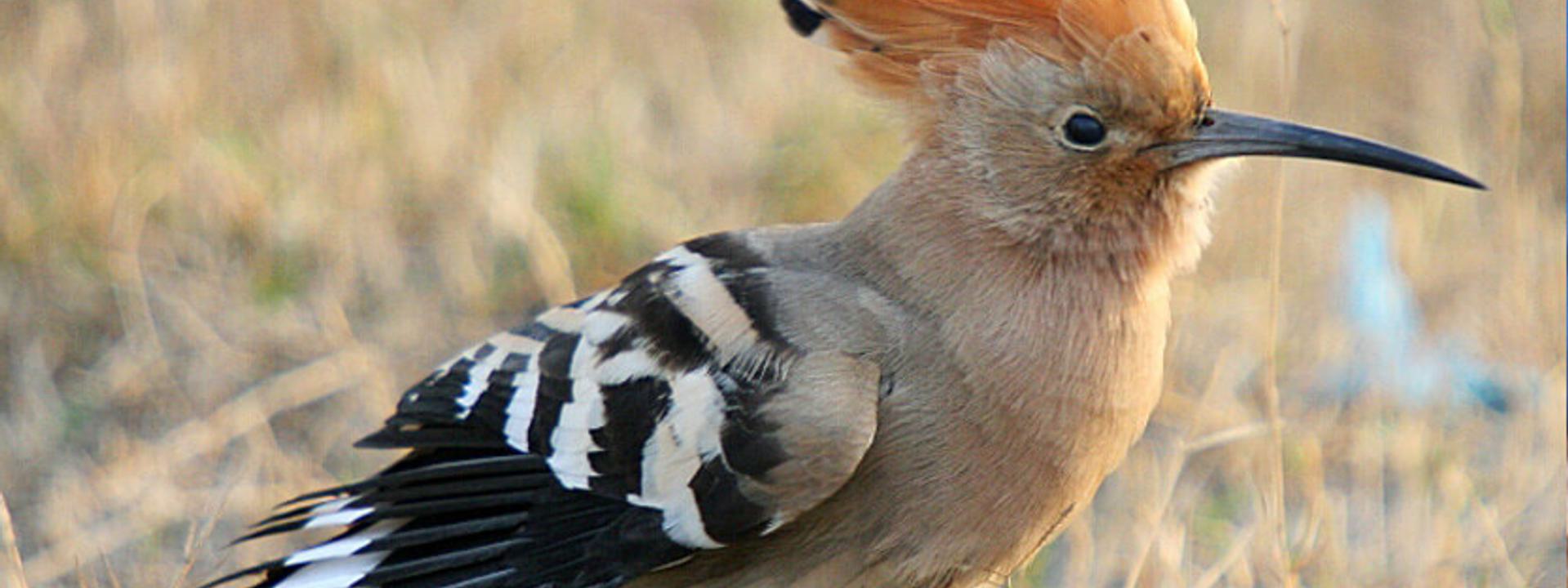In this horizontally rectangular, full-color photograph taken outdoors in a wooded setting during a day with at least some sunlight, we see a striking close-up of an exotic bird, sharply in focus against an out-of-focus background of dried, straw-like grass. The bird is depicted in profile, facing towards the right-hand side of the image.

This avian subject features a very long and thin gray beak, distinguished by its sharpness. Its vivid black eyes stand out on its head, which sports a patch of orange feathers on top transitioning to a lighter brown color beneath the bill. The bird's breast continues this light brown coloring, gradually giving way to a lighter gray body. The wings are marked with black and white stripes, and its tail feathers also exhibit a black and white pattern. Part of the bird’s feet are not visible, and the top of its head is slightly cut off by the photo. Despite the cut-off, the bird’s vibrant, detailed plumage and captivating colors make for an enchanting and beautiful subject, though the species remains unidentified. There is no text overlay to distract from this natural scene.